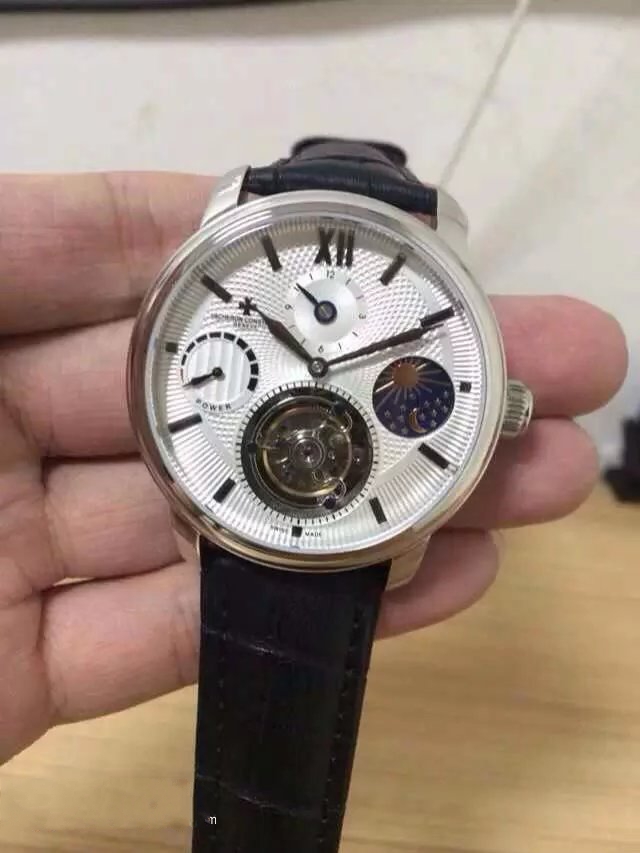A color photograph captures a close-up of a left hand, likely belonging to a white person, holding an analog wristwatch across the index, middle, ring, and pinky fingers. The backdrop features a light brown wooden surface and a white wall. The timepiece has a black leather strap, with the round face of the watch framed by a silver rim. The shimmery white face is detailed with black Roman numerals at 12 (XII) and black rectangular markers instead of numerals. Intricately designed, the watch face includes four additional sub-dials: a white top dial marked with 12, 3, 6, and 9 for months; a dial with a blue background depicting a golden sun, moon, and stars indicating day and night; a larger transparent bottom dial revealing the inner gears; and a power gauge on the left side. The main black hands of the watch point to 10:11. The detailed craftsmanship and design elements, including geometric patterns and metallic accents, underscore the watch's elegance and functionality.